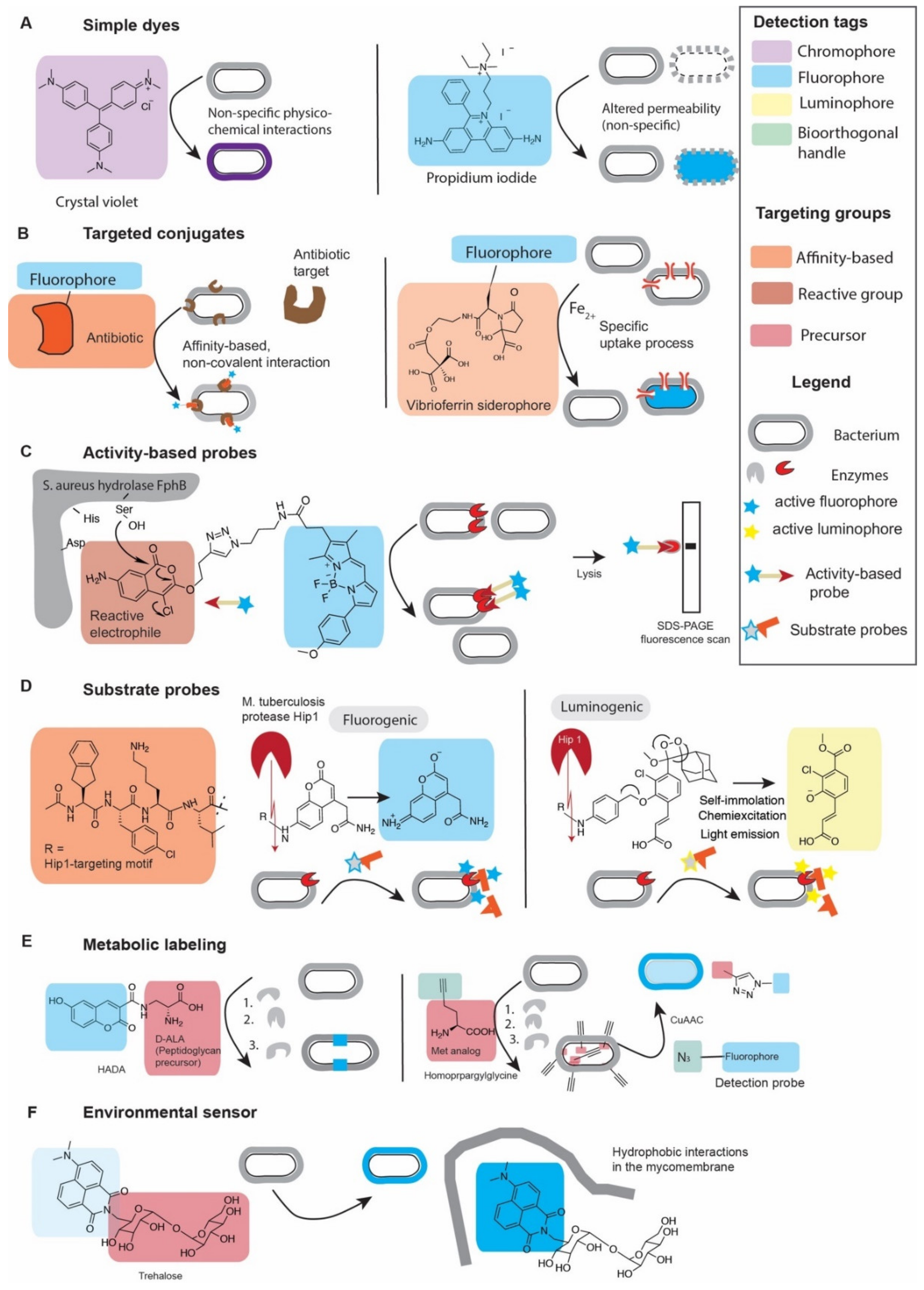This detailed and colorful science-based infographic illustrates six distinct concepts involved in various chemical processes: simple dyes, targeted conjugates, activity-based probes, substrate probes, metabolic labeling, and environmental sensors. The infographic features a complex table with a legend that decodes different colors and categories, such as detection tags and targeting groups. These tags and groups help explain processes related to bacteria, enzymes, and substrates, using both text and visual representations. On the right, a comprehensive legend provides further explanations of the colors and categories, clarifying how they correspond to different biological and chemical elements depicted in the chart. This high-quality illustration employs detailed and cartoon-like images to effectively convey the information.